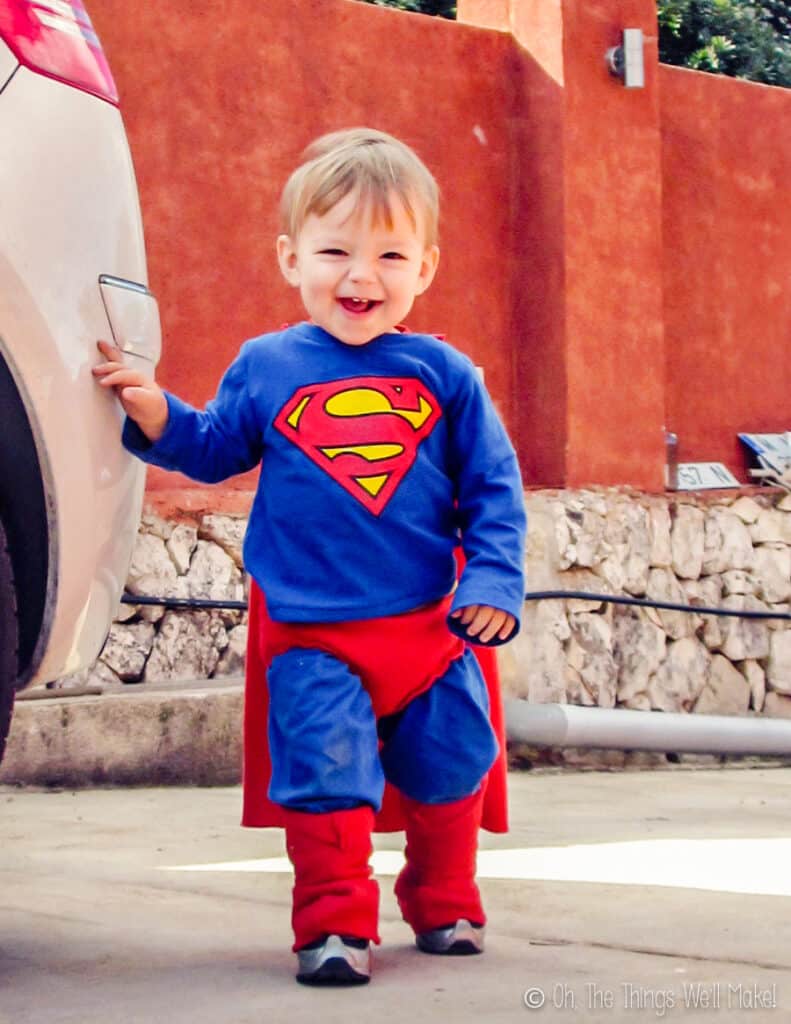This vibrant daytime photograph captures an exuberant toddler, approximately two to three years old, with short blonde hair and a wide, joyous smile on his face. He is dressed in a detailed Superman costume, featuring a blue long-sleeve t-shirt emblazoned with the iconic red and yellow 'S' logo on the chest, red briefs over blue pants, red knee-length socks over the pants, and a flowing red cape. His outfit is completed with black and gray tennis shoes. The child, of European descent, stands on a gray pavement with his right hand resting on what appears to be the rear bumper of a white vehicle, likely a minivan or crossover. 

In the background, there is a distinct two-tiered wall: the lower third is composed of a rough gray stone surface, potentially a rock face, while the upper portion is a brick-red-orange painted concrete wall. Some light fixtures and potential remnants of posters or signs are visible against the wall. The scene is bright and sunny, adding a sense of warmth and happiness to the moment captured. At the bottom right of the image, there is a copyright mark with the phrases "Oh, the things we'll make!" and "Oh, the things well done!"